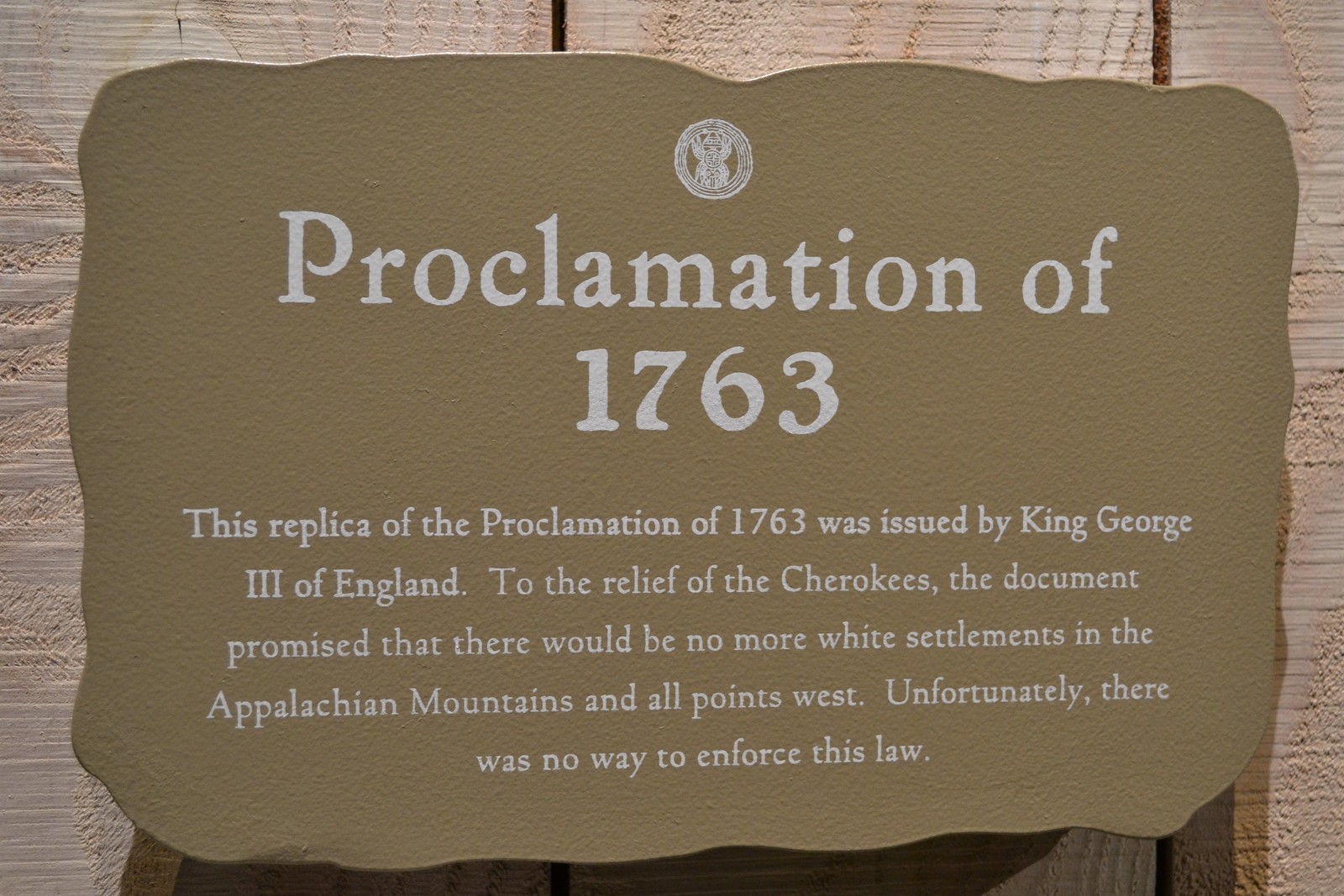The image depicts a roughly finished, light-colored wooden fence serving as the backdrop for a pale brown, cloud-shaped plaque. The plaque, attached to the wooden boards, features a circular logo at the top center, possibly including a 'B' design, although its exact meaning remains unclear. The title "Proclamation of 1763" is prominently displayed in large white letters, followed by smaller white text that reads: "This replica of the Proclamation of 1763 was issued by King George III of England. To the relief of the Cherokees, the document promised that there would be no more white settlements in the Appalachian Mountains and all points west. Unfortunately, there was no way to enforce this law." The plaque is illuminated from above and to the right, casting distinct shadows below it and slightly to the left, suggesting it projects several inches out from the wall.